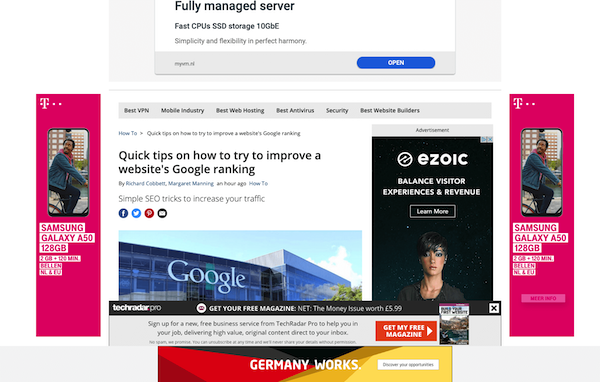At the top of the image, there is a highlighted section displaying a message that reads, "Fully managed server, fast CPUs, SSD storage, 10 GBE." The term "GBE" stands for Gigabit Ethernet. Below this, there is a tagline, "Simplicity and flexibility in perfect harmony," accompanied by a blue button with the text "Open" in white. 

On the left side of the image, the T-Mobile logo is prominently featured in the upper-left corner. Below it, a vertical banner or rectangle showcases another T-Mobile logo at the top. This banner advertises the Samsung Galaxy A50 with 128 GB of storage. The text also mentions "2 GB minimum" but the rest is indecipherable due to low resolution.

The image additionally contains a photograph of a man riding a bicycle. Alongside this photo, there are several highlighted awards or titles: "Best VPN," "Mobile Industry," "Best Web Hosting," "Best Enterprise Security," and "Best Website Builders." Below these accolades, there's a section offering tips on website optimization, including advice on improving Google ranking and enhancing web traffic. This segment is reinforced with a visual of a Google building facade, labeled with "Simple SEO tricks to increase your traffic."